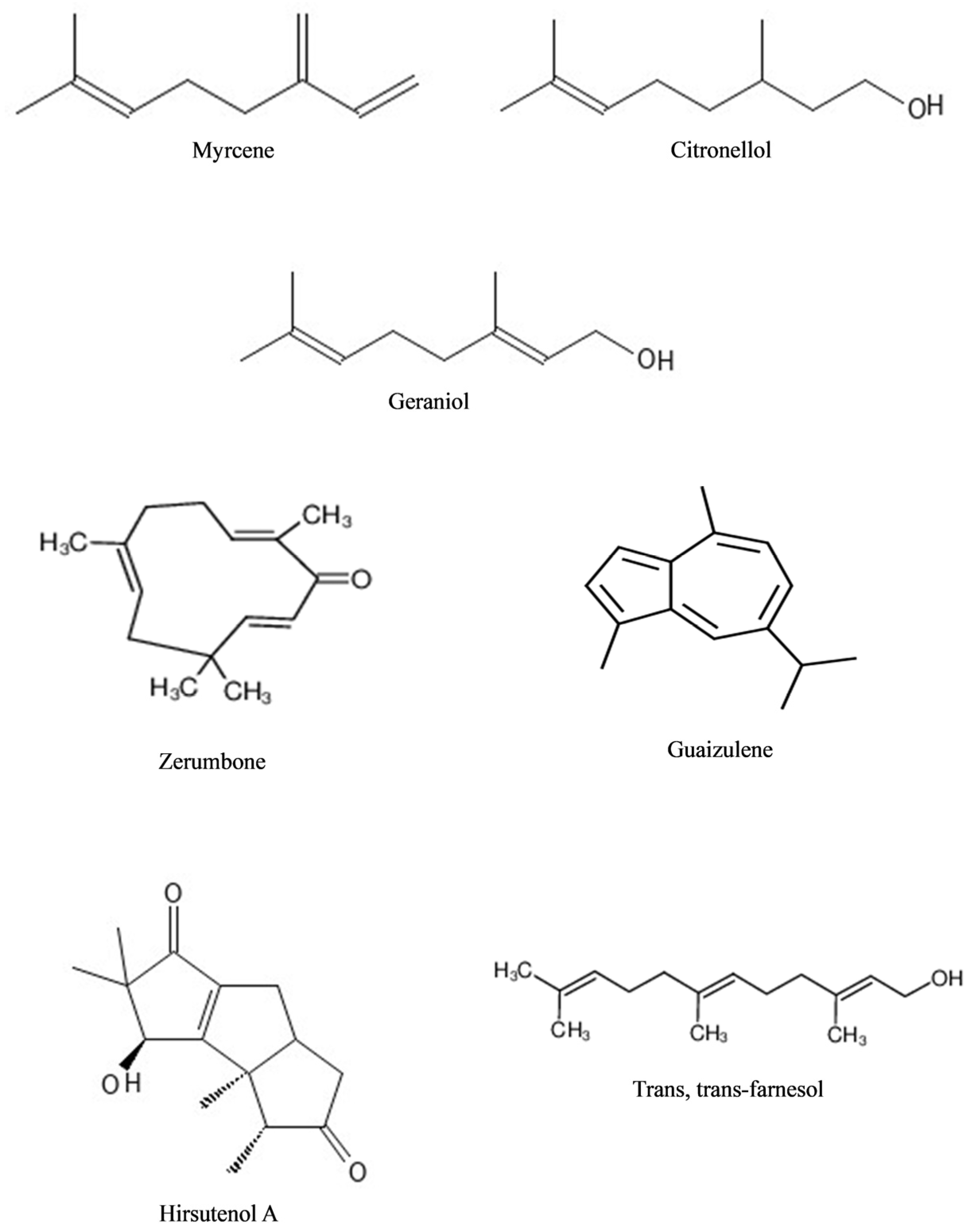The image depicts a detailed scientific line drawing commonly found in chemistry textbooks, highlighting the molecular structures of several organic compounds. Each molecule is meticulously illustrated to exhibit the arrangement of its atoms and bonds. Across the top, the drawing starts with Myserine, followed by Citronellol, both showcasing intricate carbon and hydrogen arrangements. In the center section, there is Geraniol, recognizable by its characteristic -OH group at the end. To the lower center-left, we find Xerombone, identifiable by its H3C and CH3 groups arranged in a specific pattern. Adjacent to it is Guazoline, which features two hexagon structures interconnected with various lines. Further down, on the bottom left, there's Histerly labeled with multiple hexagons and a detailed three-dimensional layout of its chemical structure. On the bottom right, the image concludes with a zigzagging Trans-Transpharmacol, marked by its alternating CH3 groups and ending with an -OH group. The entire illustration serves as a precise chemical depiction, perfect for educational purposes to show the molecular bonding and structure of these compounds.